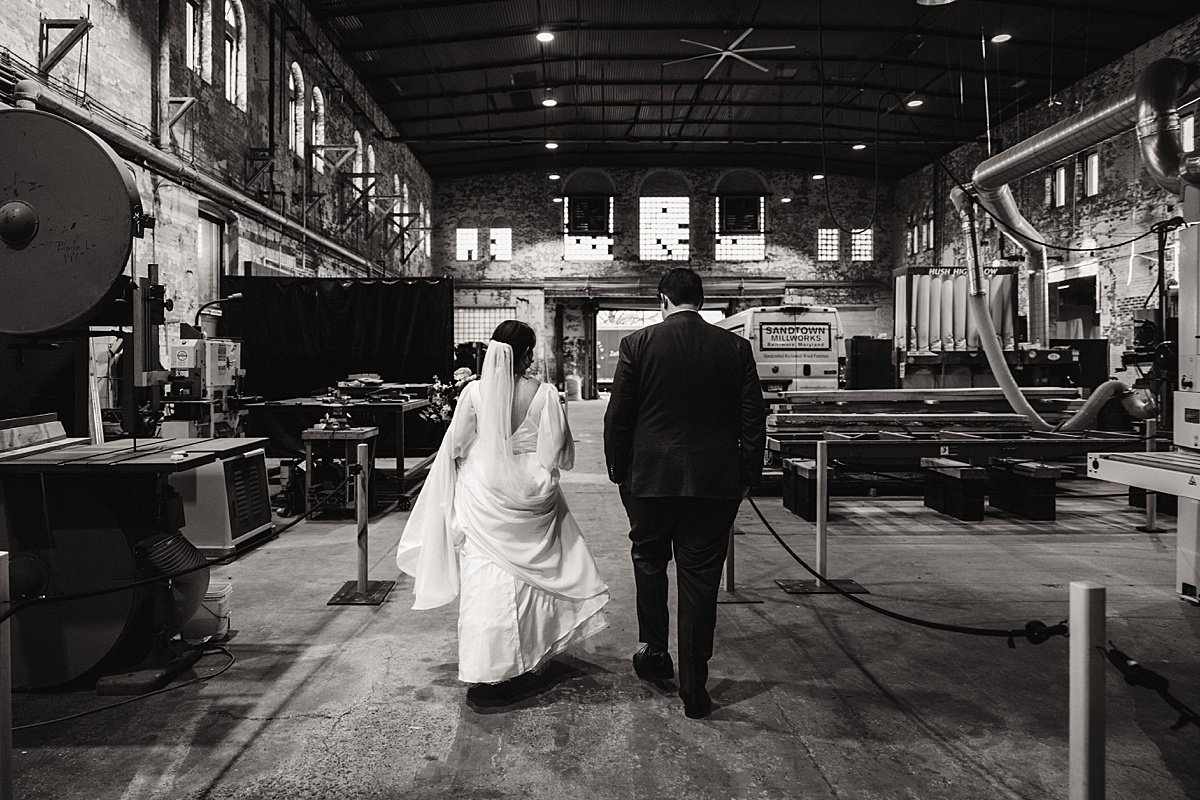In this black-and-white photograph, a bride and groom are walking hand-in-hand through a large, industrial woodworking factory with high ceilings. Their backs are turned to the camera as they move toward an entrance marked by a garage door at the far end. The bride, on the left, wears a flowing white gown with loose-fitting sleeves and a veil clipped to the back of her head, with part of the gown draped over her right hand. The groom, on the right, is dressed in an all-black suit and has his hands in his pockets. The spacious factory floor is lined with various woodworking machinery, pipes, hoses, and an iconic vehicle van bearing the logo "Sandtown Millworks." Overhead, a large industrial fan with six long blades hints at the size of the building. The couple walks through a roped-off aisle, creating a striking juxtaposition between their elegant attire and the rugged, industrial setting around them.